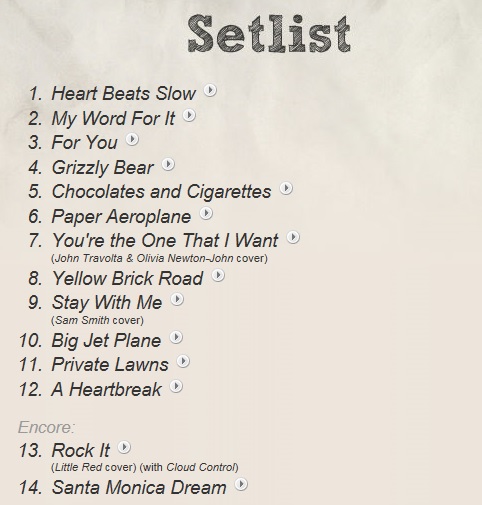The image features a digitally created graphic, resembling a piece of paper adorned with small icons, suggesting interactive elements. The background is white, and the text is black, with the title "Set List" at the top in a font that mimics pencil shading, appearing handwritten. The rest of the text is in a simple italic font, creating a clean and organized look. 

The list consists of 14 tracks, each accompanied by a small play button icon next to the track name, enhancing the modern, interactive aesthetic. The tracks are as follows: 
1. Heartbeats Slow 
2. My Work For It 
3. For You 
4. Grizzly Bear 
5. Chocolates and Cigarettes 
6. Paper Aeroplane 
7. You're the One That I Want (John Travolta and Olivia Newton-John cover) 
8. Yellow Brick Road 
9. Stay With Me (Sam Smith cover) 
10. Big Jet Plane 
11. Private Lawns 
12. A Heartbreak.

At the bottom, under the subtitle "Encore," the final two tracks are listed: 
13. Rocket, Little Red (cover with Cloud Control) 
14. Santa Monica Dream. 

The overall look of the graphic conveys a blend of traditional and modern design elements, effectively setting the mood for a curated musical experience.